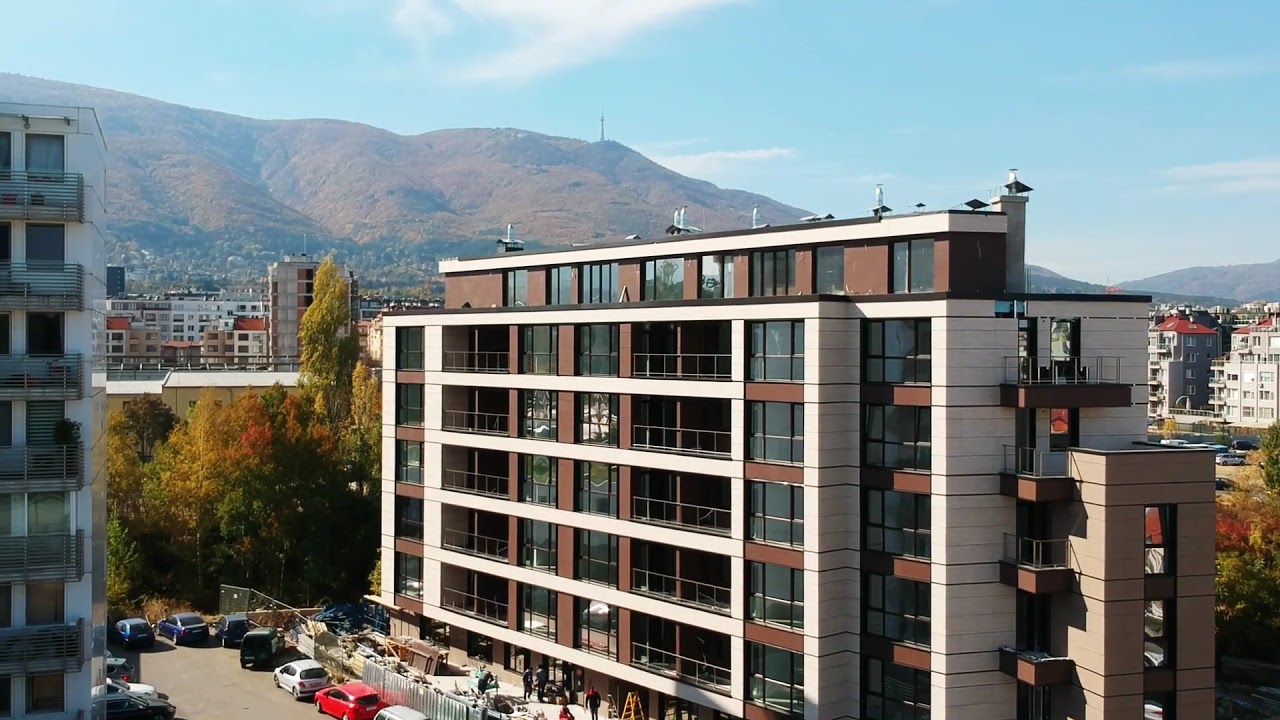The photograph captures a bustling daytime scene from an elevated position, approximately four or five stories high. Dominating the center of the image is a very tall and wide, six-story red and white building, possibly an office building, apartment complex, or medical center. This structure features numerous windows and balconies along its sides, with an additional penthouse level on top. Construction activity is visible at the building's front, where workers, a ladder, and various construction materials such as lumber and wood can be seen. The area is fenced off with a tall metal fence, and the adjacent parking lot is filled with several haphazardly parked cars.

On the left-hand side of the building, large, tall trees in vibrant shades of green, red, and gold add a natural touch to the scene. Across the street stands another six-story building with brown and off-white stonework, numerous balconies, and what appears to be an outdoor elevator. This building is directly opposite or adjacent to a taller white building with multiple balconies and stretches of other high-rise structures in the background.

The distance reveals more white buildings scattered across the town, surrounded by a picturesque brown hillside. Completing the scenic backdrop is a pale blue sky adorned with a few wispy white clouds, adding to the overall tranquil atmosphere.